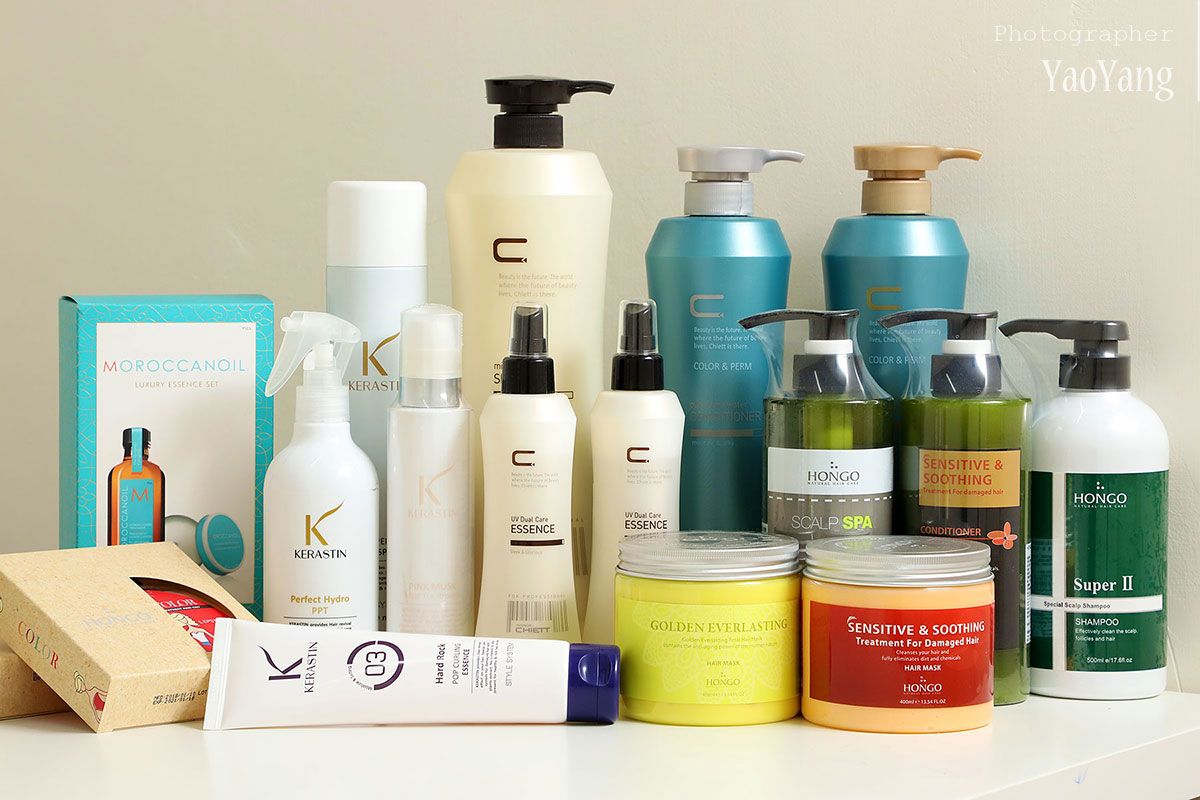In this meticulously arranged advertisement, the image showcases an array of 15 hair care products prominently displayed on a pristine white table that stretches from one edge of the frame to the other. The background is clean and white, emphasizing the products in the foreground. 

The selection includes a variety of items, with some standing tall and others lying flat with circular casing, hinting at their unique purposes. The products are aesthetically neutral in color except for two vibrant containers in the foreground, which are bright yellow and orange, labeled as Sensitive and Soothing treatments designed for damaged hair. 

Brand names such as K and C, Hongo, Moroccan Oil, and Sensitive and Soothing are clearly visible, suggesting a focus on premium hair care. Among these, specific products like Kerastin and Perfect Hydro indicate hydrating and scalp spa treatments, emphasizing the range's intent to cater to diverse hair care needs.

In the top-right corner, the name of the photographer, Yao Yang, is subtly included, lending a professional credit to the visual composition. The overall setup and clarity of the image, along with the white, uncluttered background, underline its purpose as an advertisement aimed at emphasizing the luxurious and restorative nature of the hair care products.